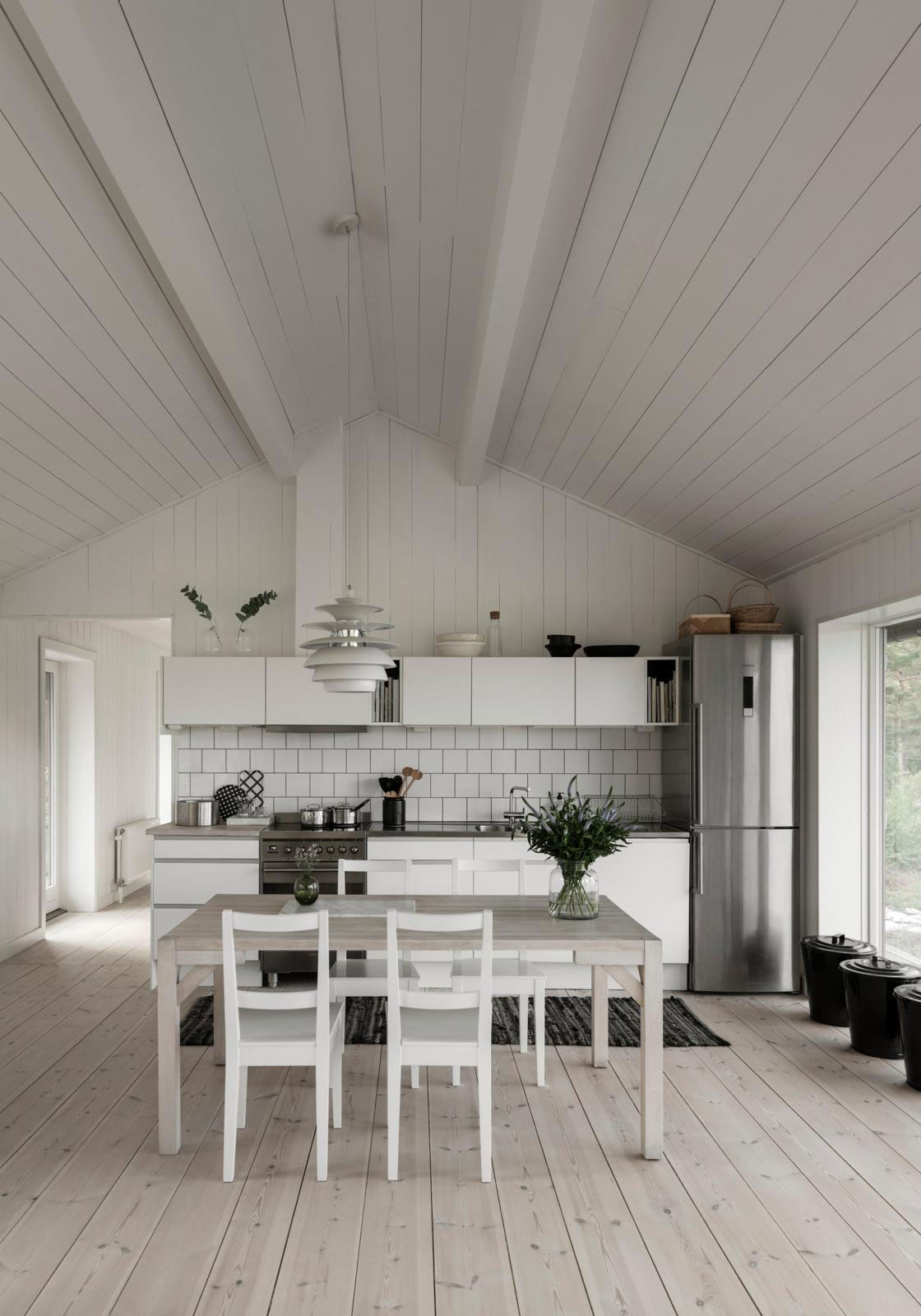This photograph captures an elegant, farmhouse-style dining room and kitchen interior, dominated by a bright white aesthetic. The room boasts very high vaulted ceilings with wooden beams and additional wooden slats arching upward, both painted white for a modern touch. The expansive space is finished with wide plank, light beige or grayish vinyl flooring that contrasts subtly with the overall white decor.

At the far end of the kitchen stands an exceptionally tall, skinny, silver refrigerator, accompanied by a standard stainless steel stove and oven, which holds a couple of pans and a black utensil holder. The kitchen cabinets are sleek and handle-free, emphasizing the minimalist design. The backsplash features a white, subway tile or exposed brick pattern, adding to the rustic yet refined look. Limited counter space accommodates only a few essential items, including perhaps a toaster and various knickknacks.

The dining area features a rectangular table with a matching wood finish akin to the floors, surrounded by four white chairs, two on each side. At the center of the table sits a circular vase filled with dried grass or dark flowers, adding a touch of natural decor. Additionally, there's a small glass on the table, contributing to the homely atmosphere.

To the right, large plate glass windows provide a glimpse of the exterior, revealing a patch of brush or a small yard. A hallway leads to other parts of the house, lined with full-length windows and featuring an old-school radiator heater. Above the oven area, shelves and drawers hold bowls and other kitchenware, while a hanging white lamp adds to the room’s cozy ambiance. The overall space exudes a warm, renovated charm, suggestive of an older home modernized with care.